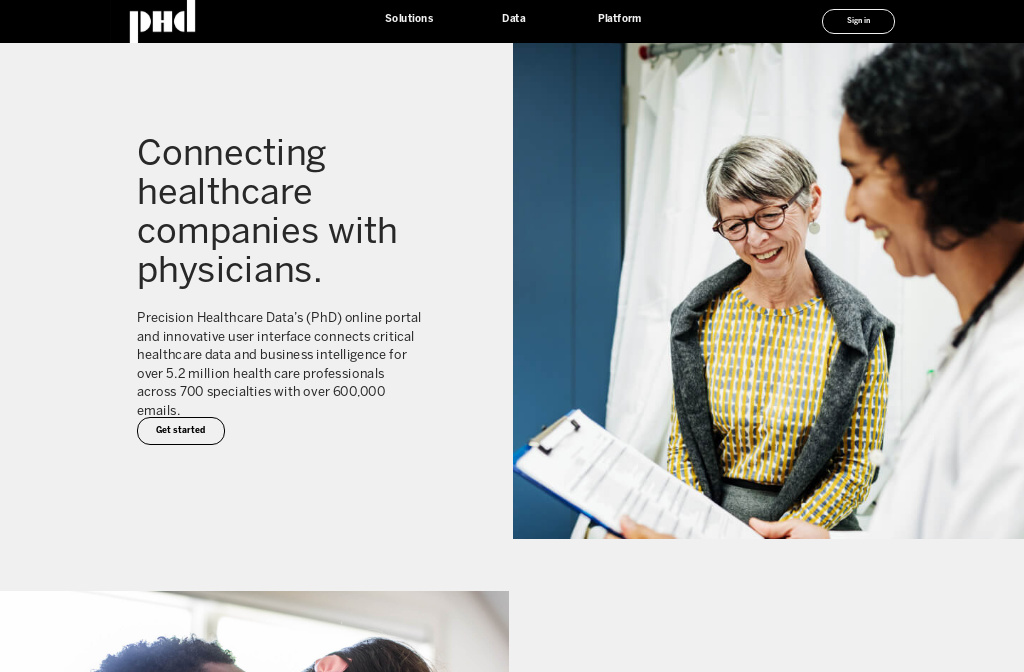The image depicts a website, likely viewed on a computer screen, showcasing a company's PhD program. The company's name and logo are positioned in the upper left-hand corner in white text on a black strip that spans the top of the page. Below this strip, the website offers solutions for data platforms and provides options to sign in, indicated by a circular icon on the right.

Prominently displayed in the center is a gray box containing a key message: "Connecting healthcare companies with physicians." This box elaborates that the "Precision Healthcare Data (PhD) online portal and innovative user interface connects critical healthcare data and business intelligence for over 5.2 million healthcare professionals across 700 specialties, with access to over 600,000 emails."

There is a call-to-action button near the bottom of this box. The button is black with white text that reads "Get Started," encircled by a black border.

On the right side of the image, there is a photograph of a woman with gray hair, dressed in a button-down shirt with a sweater draped over her shoulders. She appears to be in conversation with a dark-skinned physician, who has curly dark hair and is wearing a lab coat. The physician is holding a clipboard with a white piece of paper.

Additionally, on the left side of the screen, there is another image, though only the tops of the subjects' heads are visible, as the picture is partially cut off. Adjacent to the right of this cut-off image, there is part of a gray box positioned towards the lower section of the page.